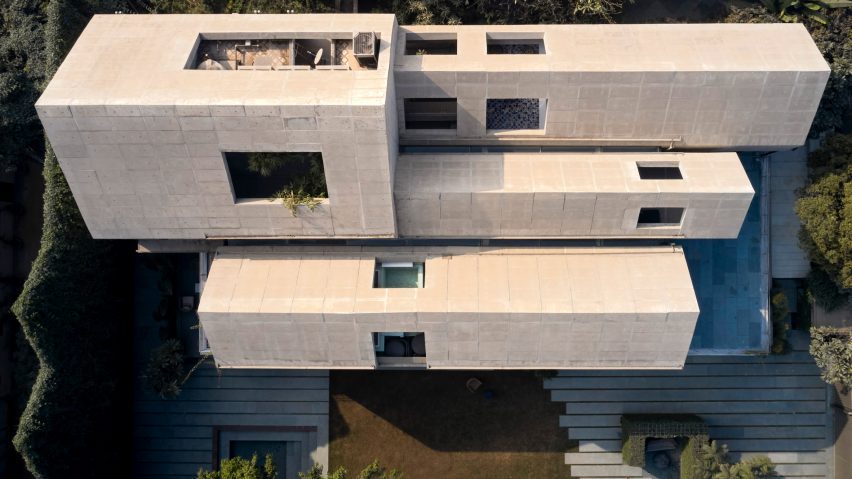This aerial color photograph, seemingly taken by a drone, showcases a modern, under-construction house characterized by its unique cube-stacked design. The architectural style resembles a three-dimensional puzzle, with the narrowest cubic structure at the bottom and progressively larger cubes stacked above. The house is primarily constructed from raw concrete or tiles, giving it a brutalist appearance. There are flat roofs throughout, punctuated by sparse windows. V-shaped roofs dominate the design, and several holes in these roofs suggest the future installation of skylights. Additionally, a long, tubular cube on the right features four windows, two on the sides and two on the top. The surrounding landscape includes visible trees and hedges, adding context to this disorienting yet striking modern architecture.